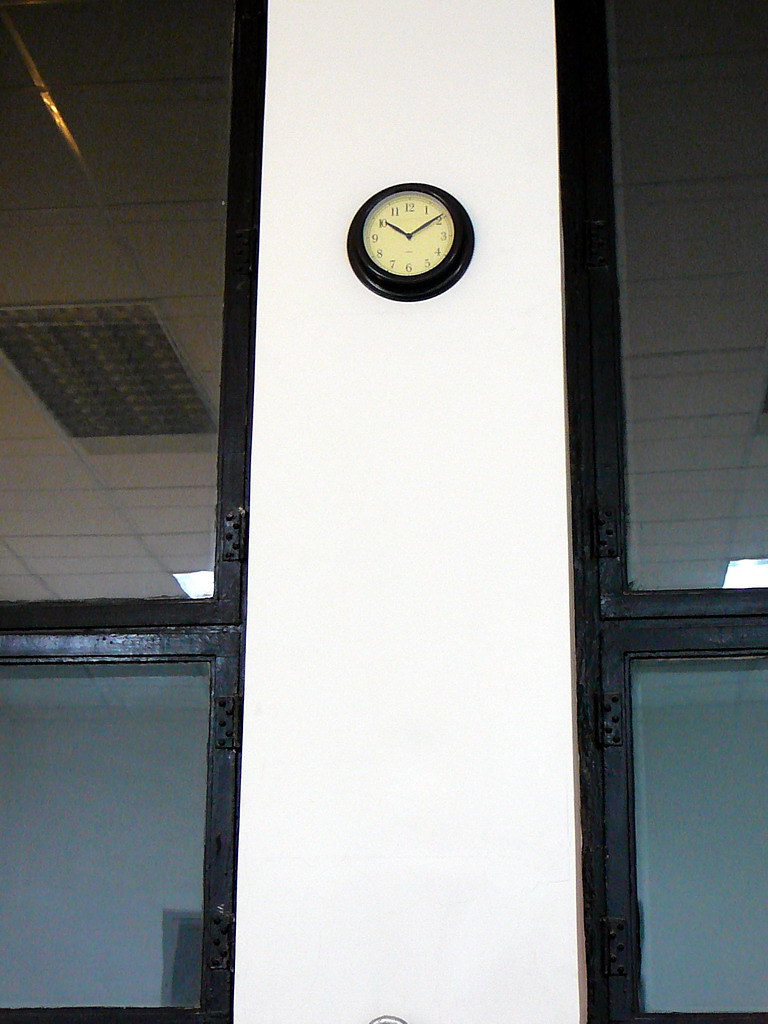The image captures a section of a building characterized by its clean, minimalist design. The white exterior wall is accentuated by black trim that frames the large windows on either side. Each window allows a glimpse into the interior, where the ceiling is lined with white tiles and features a prominent ventilation unit. A gray doorway is also visible within the building. Centrally located between the two windows on the white exterior is a sizable round black clock. The clock, featuring standard black numerals and hands, indicates the time as ten minutes past ten o'clock. Light from the interior reflects subtly on both windows, enhancing the clarity and brightness of the scene.